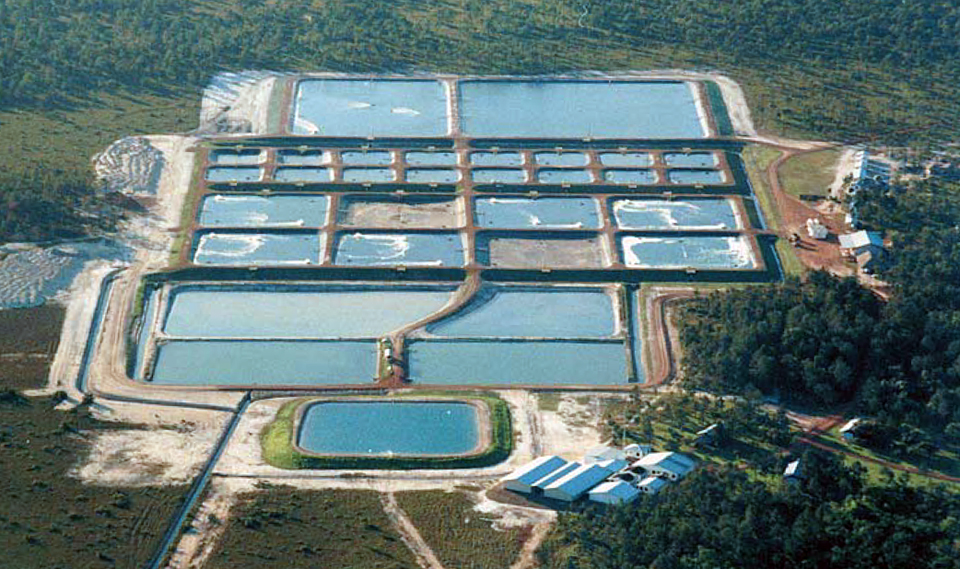This aerial image depicts a water treatment plant set in a rural area, surrounded by a tree line and expansive grassy fields. The focus of the image is a series of rectangular water treatment pools, arranged in a cascading layout from the top to the bottom of the image. The layout is as follows: 

- At the top, two large rectangular pools are situated next to each other, with the left pool being about half the size of the one on the right. 
- Below these, there are two rows of eight smaller pools.
- Directly underneath, two additional rows of four medium-sized pools each are aligned.
- Further down, near the bottom, two elongated rectangular pools stretch from left to right.
- At the very bottom, there's a final, smaller pool surrounded by green grass and sand.

Throughout the image, the pools are outlined and divided by metal structures, and the entire area is interconnected by a network of gravel roads and pathways. In the bottom right corner, several small buildings with blue and white roofs are visible, possibly maintenance or administrative structures related to the plant. The overall layout and functionality suggest the facility is dedicated to water treatment, although the possibility of it being a fish hatchery was also considered. Bartlett elaborates on details like aeration, concrete bottoms in certain ponds, and varying pool sizes which contribute to the site's infrastructure.